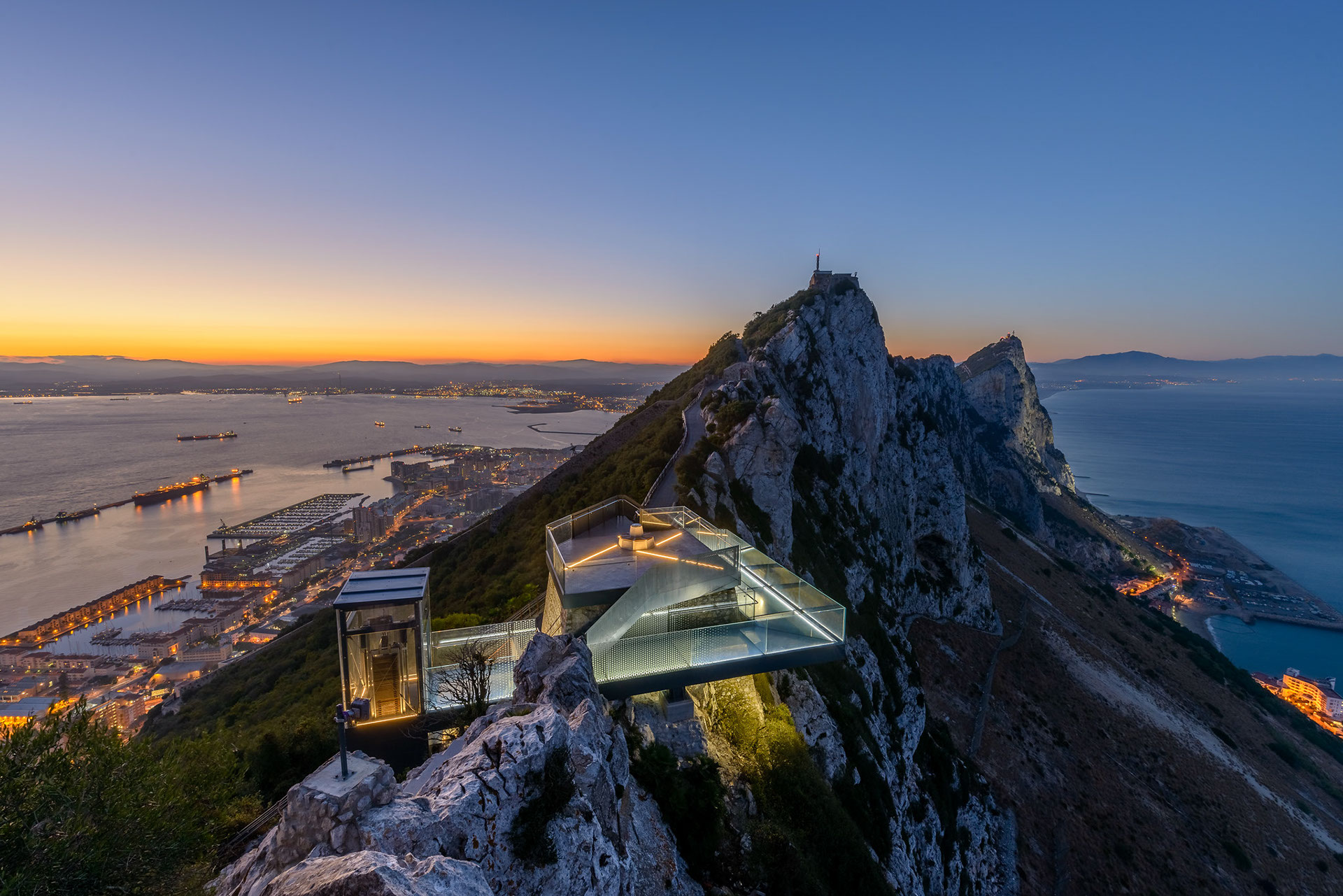This image features a striking, modern house perched on a rugged mountainside. The house, primarily constructed of glass, consists of a series of rectangular and square sections in shades of gray, yellow, and blue. One part of the house notably extends out over the cliff, emphasizing its bold, architectural design. The mountainside beneath the house is a blend of bluish-gray rock and verdant green grass, contrasting with the structure’s sleek lines.

In the foreground on the left, there is a walkway edged with glass railings connecting different parts of the house. To the right of the house, the mountain transitions from a light gray to a light brown hue with a noticeable gray streak.

Beyond the cliff, the expansive view reveals a vast ocean with a mix of dark and light blue waters, seamlessly blending into the horizon. On the left, docks stretch into the water, hinting at nearby human habitation. The distant skyline illustrates a captivating sunset, painting the sky in vibrant shades of orange, yellow, pink, and blue. Below the colorful expanse, a shoreline city glimmers with lit-up buildings, adding a sense of liveliness and contrast to the serene natural setting.